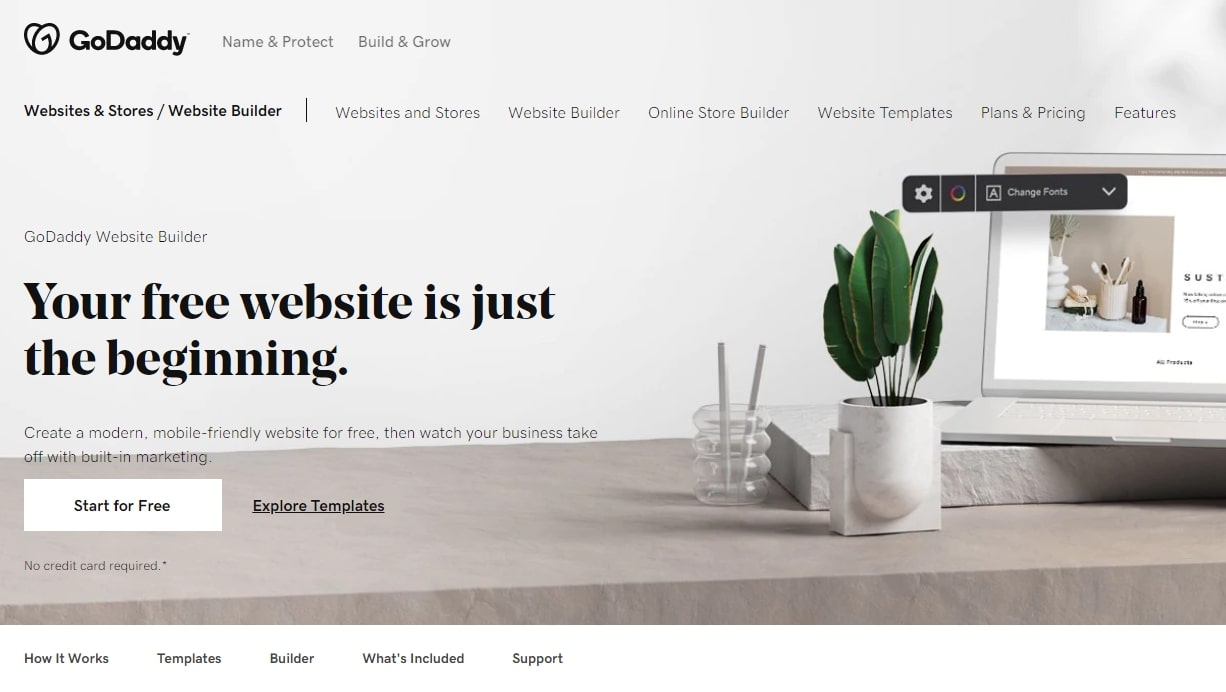The illustration features a gradient gray background that transitions from darker at the top to lighter at the bottom, giving the impression of a sleek and modern desktop setup. Positioned on the right-hand side of the desk is a laptop computer, emblematic of a workspace. To its left, a unique container resembling a cup is brimming with greenery; it could serve dual purposes, either as a plant pot or a decorative pencil holder.

In the upper left corner of the image, we see the distinctive GoDaddy logo. The logo comprises an abstract shape paired with the company name "GoDaddy" written boldly next to it. Adjacent to the logo are several lines of text rendered in various shades of gray. The first set of words in light gray is followed by another set in darker gray text, separated by a slash. This text sequence is underscored by a horizontal line, leading into more gray text that stretches until the right edge.

On the right side of the layout, there is a black, rectangular area with smooth, curved corners. This section contains several graphical elements: a gear shift icon, a multicolored line forming a circle, a white line, a square shape with additional details, accompanied by text and a downward-pointing arrow.

Beneath these icons, a phrase reads, "Your free website is just the beginning," followed by additional lines of text. Dominating the lower section is a prominent white rectangle bearing the call-to-action "Start for free." Below this button, more underlined text is placed, written in brown, adding to the call-to-action sequence.

Finally, surrounding the central visual elements, there are supplementary textual details aligning to the left and right of the image, contributing to the overall narrative and guiding the viewer through the visual content effectively.